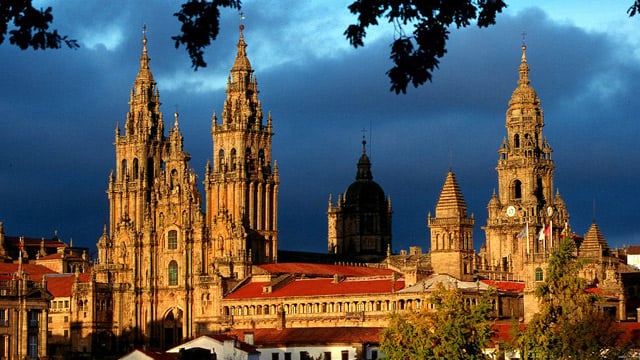The color photograph captures the majestic Cathedral of Santiago in Spain at dusk, set against a dark blue sky with ominous gray clouds. The landscape-oriented photo highlights the cathedral's elaborate architectural features, including its tall towers, pointed spires, and red-tiled roofs. The central part of the structure boasts a low, expansive section with vibrant red tiles, flanked by several towering spires on the left. Additional red-tiled sections and shorter towers with pinnacles adorn both sides of the cathedral. The right side reveals a domed structure silhouetted against the dimming light. The scene is accentuated by the castle being illuminated, creating a stark contrast with the surrounding trees and darkened sky. Stained glass windows glimmer, and flags can be spotted flying on both the right and left sides of the image. The composition beautifully showcases the grandeur and intricate details of the cathedral's design, evoking a sense of historical splendor and architectural mastery.